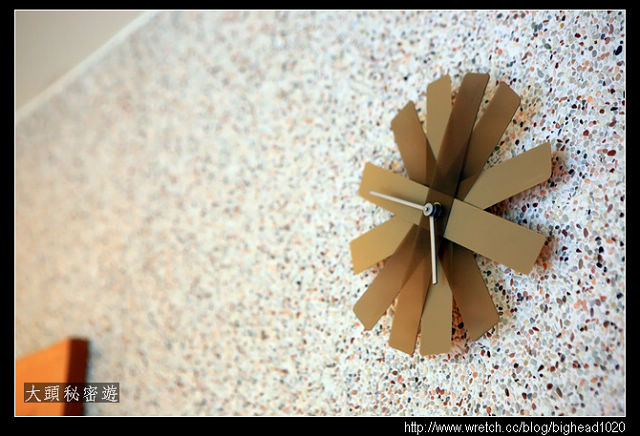This photograph features a unique wall clock made of rectangular strips, reminiscent of plastic or Popsicle sticks, arranged in a radial pattern to form a snowflake-like structure. The clock showcases various shades of tan and brown, including dark and milk chocolate hues, with hands indicating the time around 10 to 6. Mounted on a marbled wall or surface with specks of maroon, orange, black, light brown, olive green, and blue, this clock is both intricate and colorful. In the lower left corner of the image, there is an orange poster accompanied by some Asian script, likely Chinese or Japanese, adding a cultural touch to the scene. Additionally, the bottom right corner contains a website address, http://www.wretch.cc/blog/bighead1020, set against a black border, though it is somewhat blurred and hard to read.